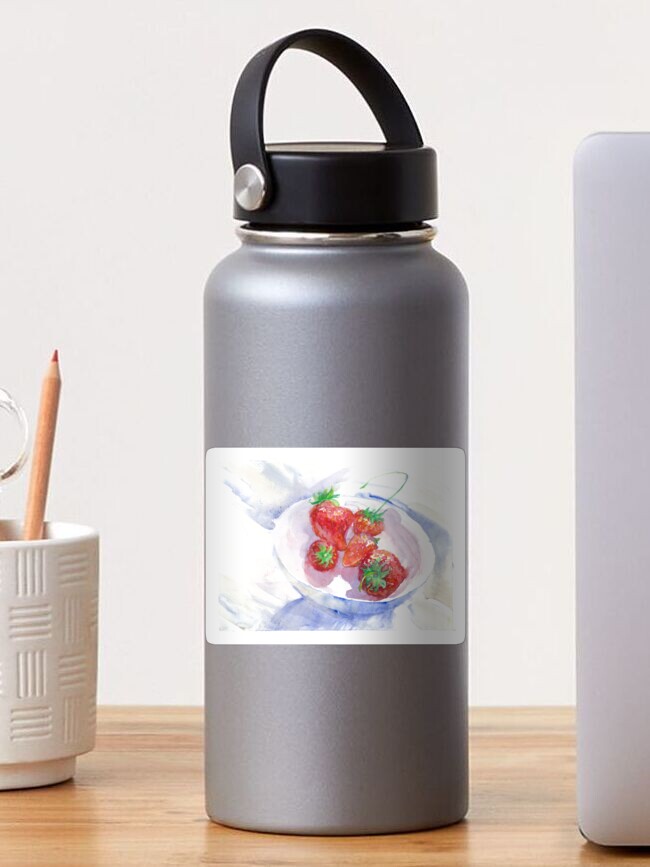The image depicts a neatly arranged workspace, with a central focus on a silver water bottle. The bottle, likely metal with a powder-coated finish, features a black screw-off lid with an attached black handle. The bottle bears a graphic that appears to be a digitally inserted hand-drawn illustration of bright red strawberries in a white bowl with a hint of blue. This graphic suggests the image might be a demo photo typically used by sellers of customizable merchandise, like stickers or t-shirts, where different graphics can be overlaid depending on the context.

On the right side of the image, the edge of an open silvery laptop is visible, as though viewed from behind, with its screen not in the line of sight. The wooden desk supporting the items is a light, blonde color, adding a natural touch to the setup. To the left, there is a cup containing a colored pencil and possibly a pair of scissors, hinting at a creative or work-related environment. The background features a white or off-white wall, ensuring that the focus remains on the items in the foreground.